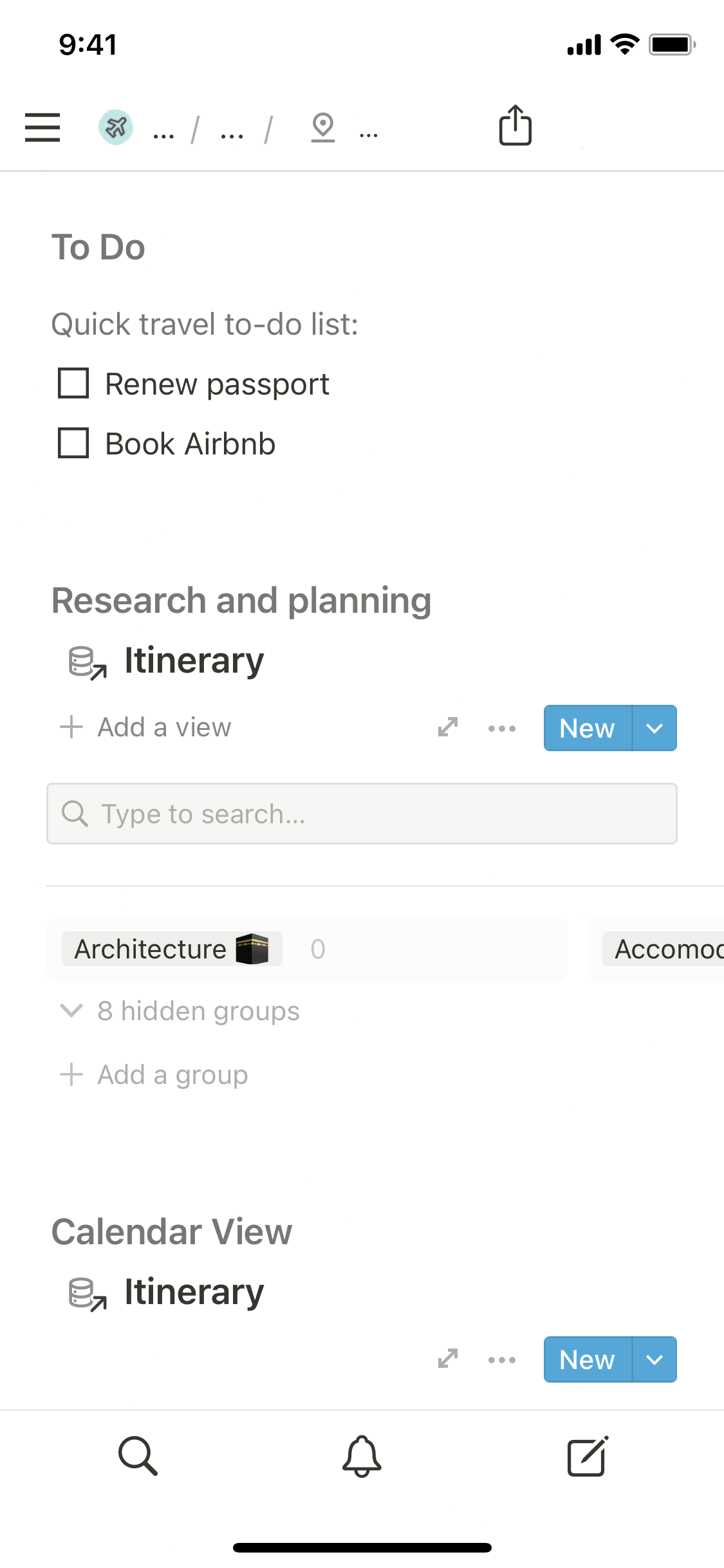A detailed caption for the given image:

"This screenshot, taken at 9:41 as indicated by the time display in the top-left corner, showcases a planning application interface. On the top-right, there are icons displaying the current cellular data signal, Wi-Fi signal, and battery level. The main section below features a categorized to-do list, beginning with a 'Quick Travel To-Do List' that includes tasks such as 'Renew Passport' and 'Book Airbnb,' each accompanied by a checkbox. The subsequent section is titled 'Research and Planning,' featuring an option labeled 'Itinerary' and a button beside it allowing users to add a new view. To the right of this, a 'New' button and a search bar are conveniently placed for easy navigation. Further down, the 'Architecture' section follows with a note about eight hidden groups and an option to add a new group. The final section at the bottom is labeled 'Calendar View,' also related to an 'Itinerary,' ensuring users can manage their travel plans efficiently."